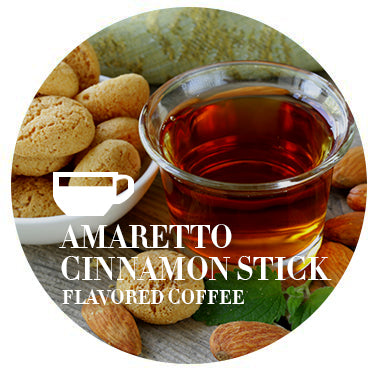The circular advertisement image showcases a clear glass of lightly brewed Amaretto cinnamon stick flavored coffee, resembling tea, and topped with a flared rim. Surrounding the coffee on a table are assorted biscuits, including Amaretto cookies and almonds, along with an herb leaf, possibly mint. A white ceramic dish filled with more biscuits accompanies the setup. The background features a seafoam green wall, adding a soothing touch to the scene. Overlaying the image is white text in a serif-type font, stating "Amaretto cinnamon stick flavored coffee," accompanied by a white logo of a coffee mug, three-quarters filled, positioned above the text.